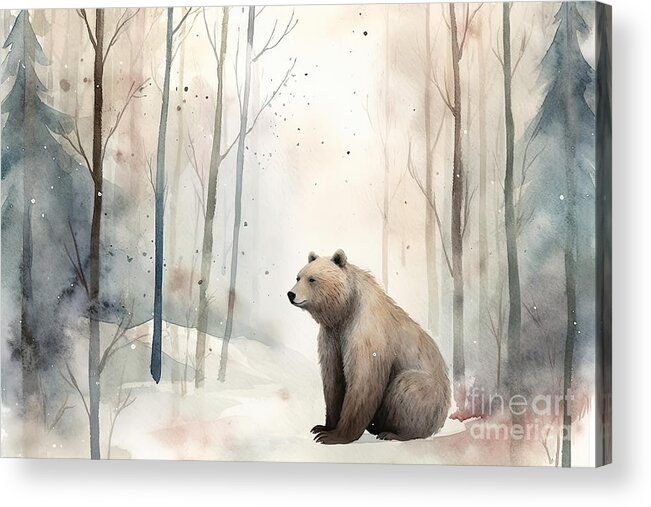The image depicts a detailed, artistic painting of a large, realistic brown bear, sitting on its hind legs amidst a wintry, forested landscape. The scenery is abstract and features a frozen creek surrounded by sweeping banks, with bare trees and dark evergreens in the background. Bright reflections of light illuminate the snowy surroundings, enhancing the impression of a cold, winter day. The bear appears almost superimposed onto the scene, strikingly rendered with lifelike detail compared to the more splotchy, watercolor-like background. Fine Art America’s watermark is visible in the bottom right corner of the image.